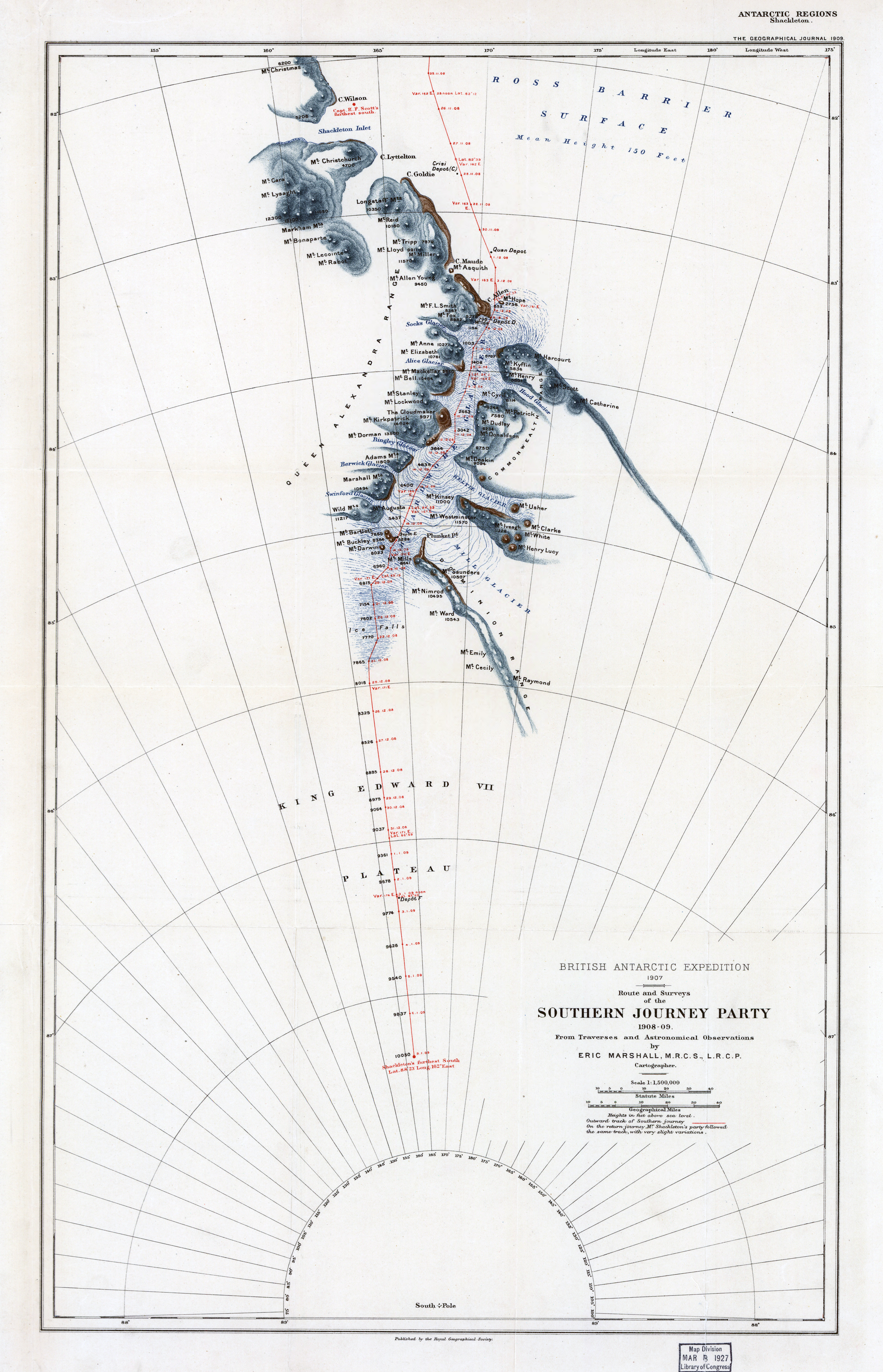The image depicts a detailed map labeled "Antarctic Regions" at the top, showcasing the geographical layout of parts of Antarctica. Prominently featured in the upper section of the map is the "Ross Barrier Surface," indicating a significant landmark in the area. Although many of the landscape names on the map are too blurred and small to decipher, the bottom of the map distinctly reads "British Antarctic Expedition," likely dated to 1997 in very small font. The map also prominently highlights "Southern Journey Party" in bold print, documenting the expedition period from 1908 to 1909. Additionally, the name "Eric Marshall" is visible, along with his credentials "MRCS LRCP," suggesting his involvement in the expedition.